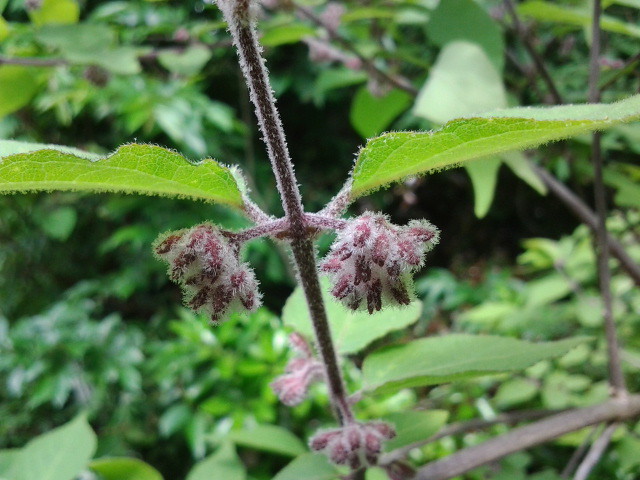This image is an outdoor photograph taken in a naturally bright yet cool light setting, likely in a wooded area or garden. The background is a lush, vibrant green mass of various types of foliage, slightly blurred to draw attention to the main subject. Prominently featured in the foreground is a singular stem, tilted at a slight angle. The stem, a dark red or burgundy color, is densely covered with fuzzy white hairs. From this stem, two large leaves extend, also enveloped in fuzzy, hair-like structures, reminiscent of tiny spider hairs.

Additionally, the stem bears four cluster-like structures hanging down, which may be flowers or seed pods. Each of these clusters is similarly adorned with the same fuzzy, white coating, giving them a somewhat bulbous appearance. Within these clusters, individual seeds or tiny blossoms can be discerned, tinged with a subtle purple hue. They create a striking focal point amidst the sea of greenery, all of which appears healthy and vibrant, indicating a thriving natural environment.